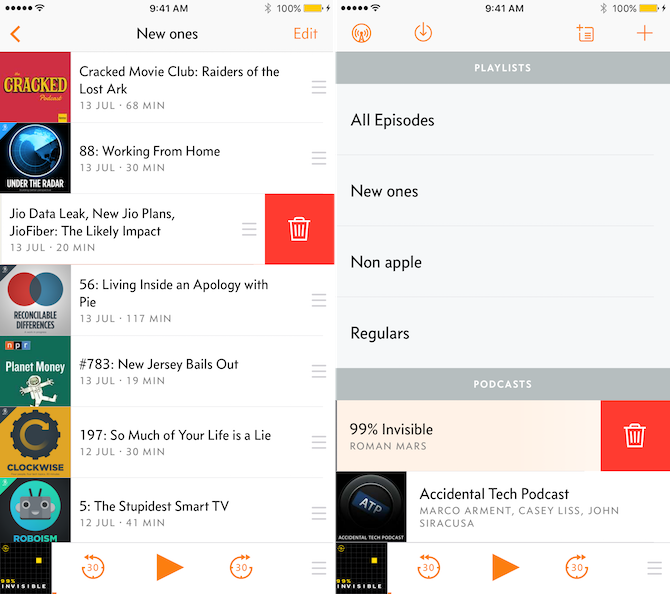The image consists of two side-by-side screenshots. 

On the left side, the screenshot features a digital interface displaying a list of media items. The top of this screenshot indicates the time as "9:41 AM" in the top-left corner, with the label "New Ones" in black beneath it. Positioned vertically along the left side are thumbnails, which likely represent book covers or podcast thumbnails, accompanied by their titles in black text. The list includes:
1. "Cracked Movie Club" followed by "Raiders of the Lost Ark," dated "13 July" with a duration of "68 minutes."
2. "Working From Home" from "13th of July," lasting "30 minutes."
3. An entry with no thumbnail titled "JIO Data Leak, New JIO Plans, JIO Fiber, The Likely Impact," which features a trash can icon on its right side.
The list continues with:
4. "Living Inside an Apology with Pi" numbered "783."
5. "New Jersey Bails Out" with "197."
6. "So Much of Your Life is a Lie."
7. "The Stupidest Smart TV."

The right side screenshot is labeled "Playlist" at the top. Below it, in black text, are the categories: "All Episodes," "New Ones," "Non-Apple," and "Regulars." A gray bar below these categories, labeled "Podcasts" in white text, lists:
1. "99% Invisible" by Roman Mars, with a trash can icon next to it.
2. "Accidental Tech Podcast."

This detailed and organized caption provides a clear description of the elements within the dual-screenshot image.